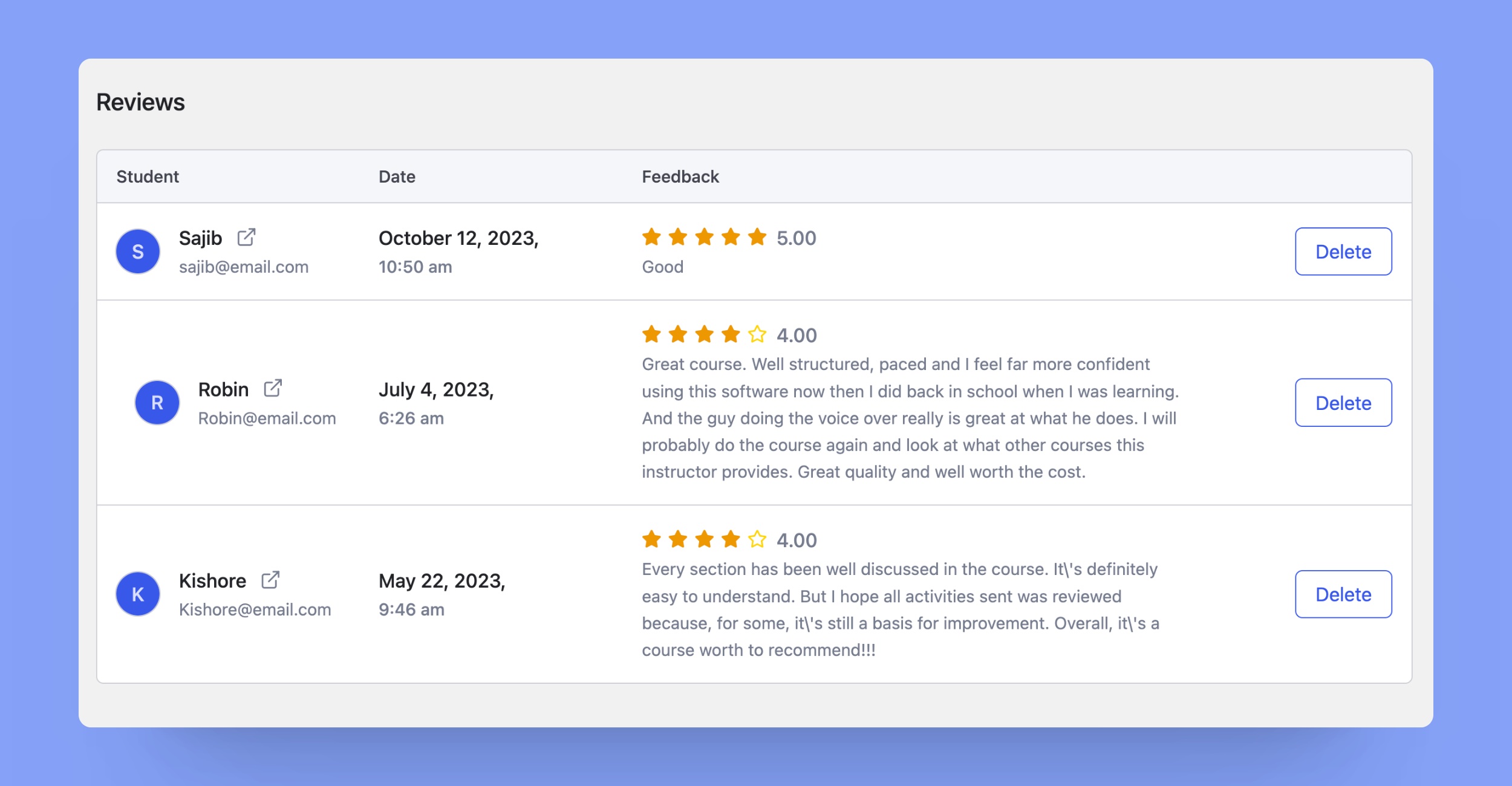The image displays a screenshot cropped from a review site, specifically geared towards academic courses. In the top left corner, the word "Reviews" is prominently featured, indicating the focus of the content. Below this heading, there are three columns labeled "Student," "Date," and "Feedback."

1. **Student: Sajib** - **Date: October 2023** 
   - **Rating: 5 Stars** 
   - **Feedback: "Good."**
   - Sajib succinctly expresses satisfaction with the course, awarding it the highest rating of five stars.

2. **Student: Robin** - **Date: July 2023**
   - **Rating: 4 Stars**
   - **Feedback: "Great course, well-structured, and paced. I feel far more confident using the software now than I did back in school when I was learning. Great quality and well worth the cost."**
   - Robin praises the course’s structure and pacing, highlighting an increased confidence in using the software and deeming the course a worthwhile investment.

3. **Student: Kishore** - **Date: May 2023**
   - **Rating: 4 Stars**
   - **Feedback: "Every section has been a little discussed in the course. It's definitely easy to understand, but I hope all activities sent were reviewed, because for some, it's still a basis for improvement."**
   - Kishore appreciates the course’s ease of understanding, though suggests that there might be room for improvement in the review of certain activities.

Each review is recent, with Sajib's being the most updated in October 2023, followed by Robin's in July 2023, and Kishore's in May 2023. Collectively, the feedback indicates a high level of satisfaction among the students.